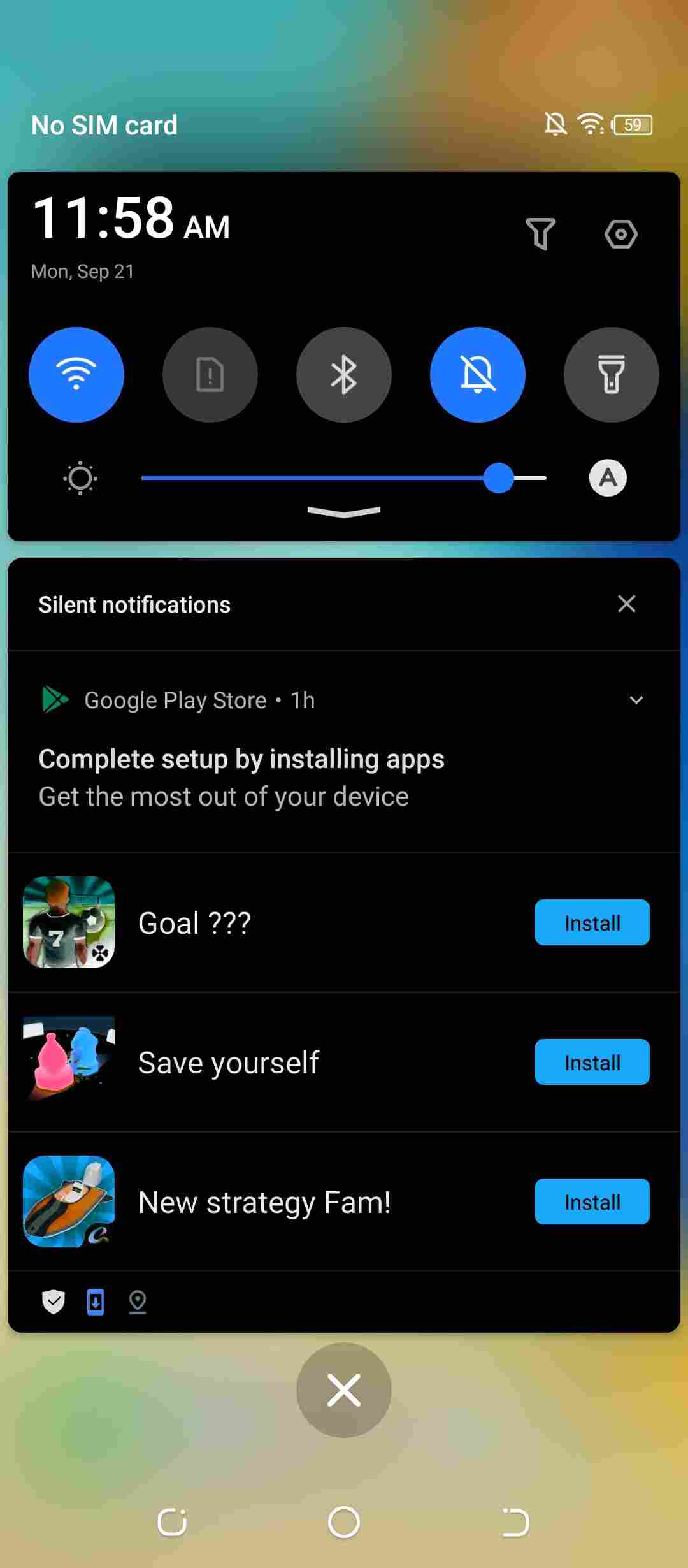This image depicts a smartphone against a colorful, blurred background featuring shades of green, brown, and yellow. In the top-left corner of the display, the message "No SIM card" is visible. On the top-right, several icons are present: a notification bell, a disabled WiFi symbol, and a battery indicator showing 59% remaining. Below these indicators is a black panel displaying the time, 11:58 AM, on the left-hand side. Also visible on this panel are greyed-out icons for Bluetooth and a torch, alongside active icons for WiFi and notifications.

Additionally, there is a brightness control slider positioned under this section. Below that is a "Silent notifications" option marked by an X. Further down, the Google Play Store is open, prompting the user to complete the setup by installing apps. Three suggested apps are listed for installation: "Goal ???" with an install button in blue, "Save Yourself" with a corresponding install button, and "New Strategy Fam!" also featuring a blue install button.